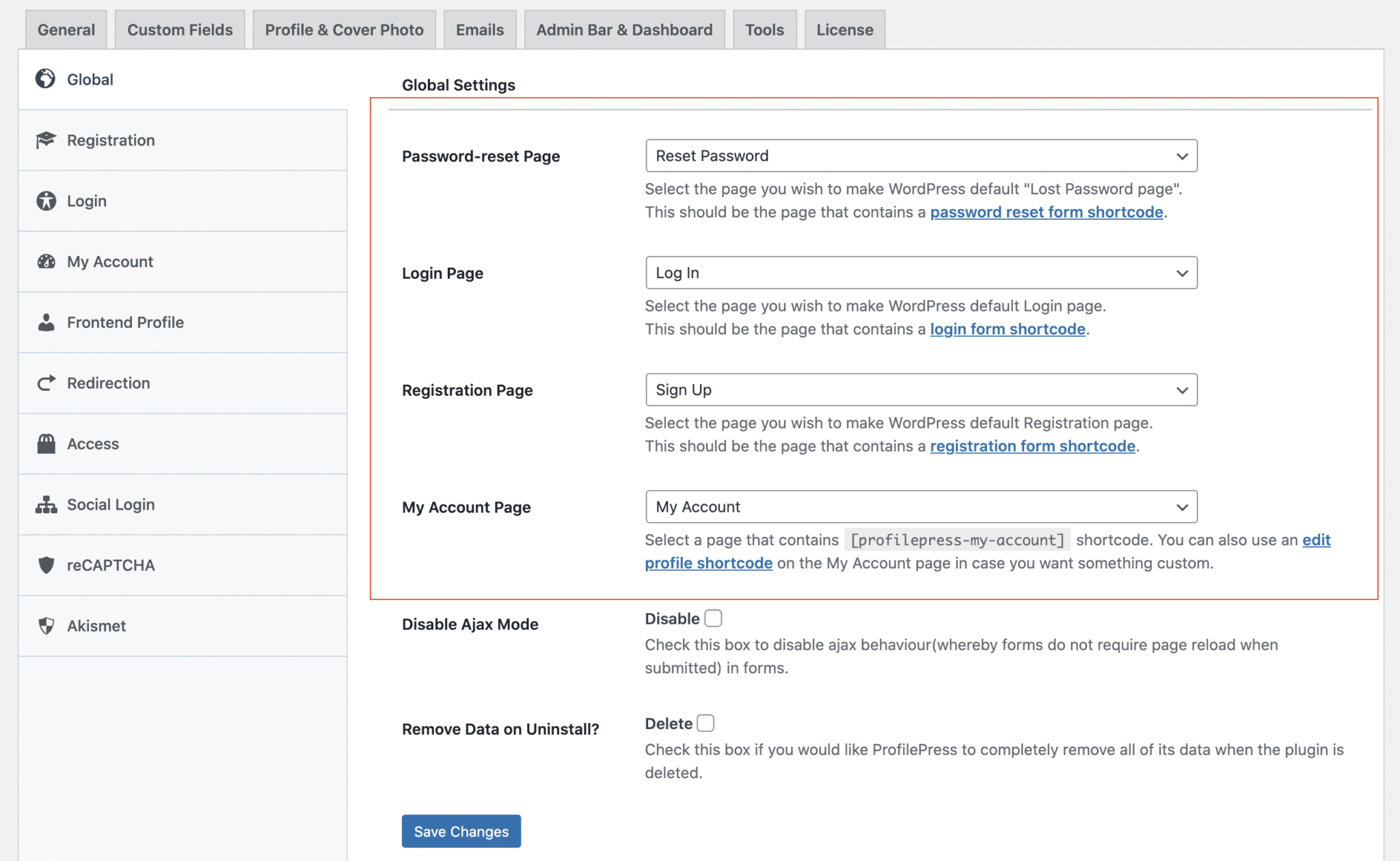The image depicts a screenshot of a settings interface from a software application on a computer screen with a white background. At the top of the window, there is a row of gray tabs labeled from left to right as follows: General, Custom Fields, Profile and Cover Photo, Emails, Admin Bar and Dashboard, Tools, and License.

On the left side of the interface, there is a vertical menu labeled “Global” at the top. Below this label are more sub-categories listed sequentially: Registration, Login, My Account, Front End, Profile, Redirection, Access, Social Login, ReCAPTCHA, and Akismet.

To the right of this vertical menu, the main content area presents a section titled "Global Settings." Within this section, there is a rectangle outlined in red containing several dropdown options:

1. **Password Reset Page:** Accompanied by a dropdown menu currently set to a reset password page.
2. **Login Page:** Accompanied by a dropdown menu currently indicating "Login."
3. **Registration Page:** Accompanied by a dropdown menu currently set to "Sign Up."
4. **My Account Page:** Accompanied by a dropdown menu currently set to "My Account."

Below this red-outlined rectangle are additional settings with checkboxes:

- **Disable AJAX Mode:** An option with an associated checkbox, which is currently unchecked.
- **Remove Data on Uninstall:** Another setting with a checkbox, which is also currently unchecked.

At the very bottom of the interface is a blue button labeled "Save Changes."